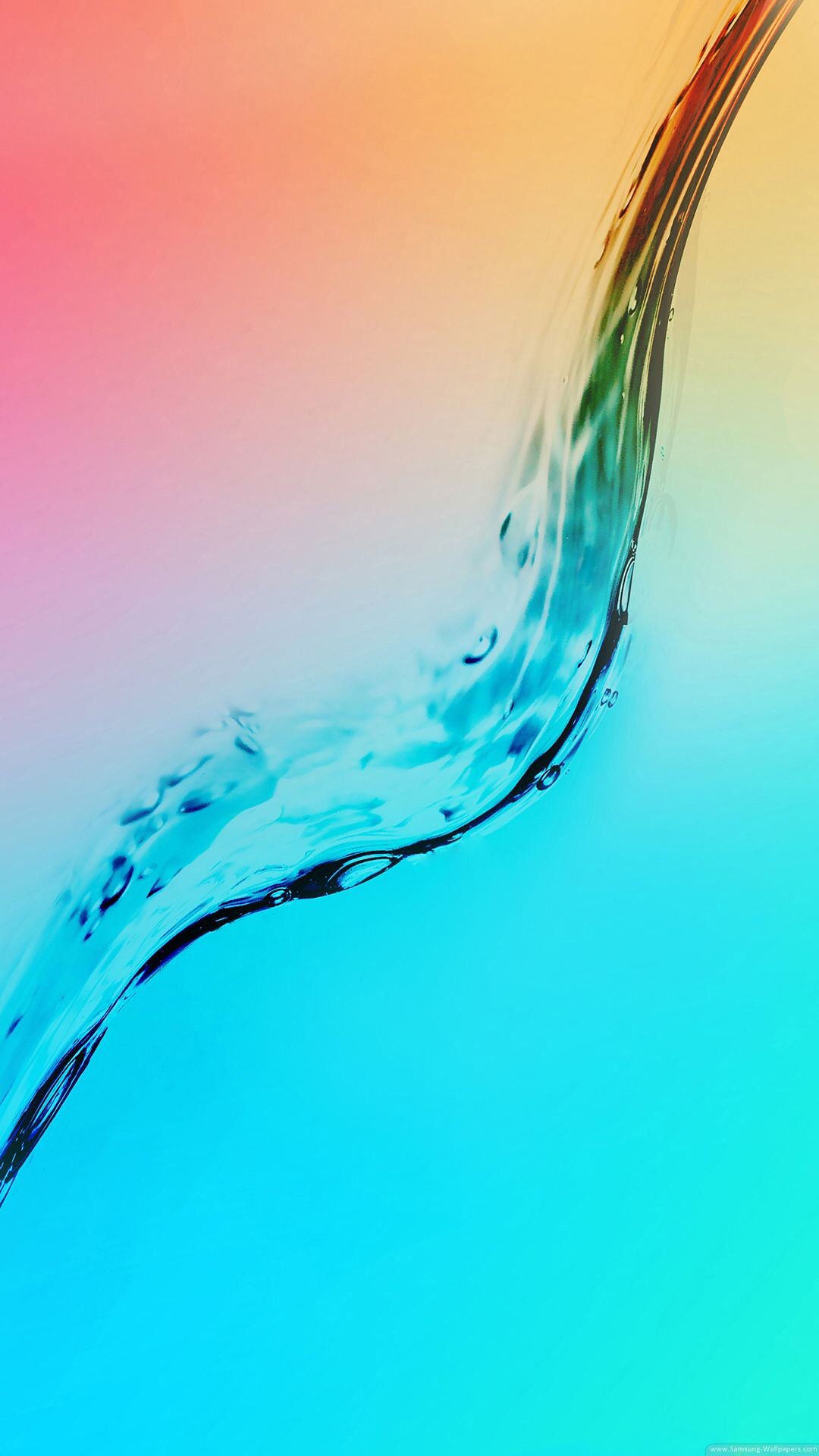The image appears to depict a vertical rectangular graphic with a gradient background that transitions smoothly through a spectrum of colors. Starting from the top left corner, it showcases a warm peachy rose hue that changes to orangish-yellow at the top right. Moving downwards, the gradient flows into soft yellows, then transitions to an aqua blue that evolves into a teal and turquoise palette towards the bottom right, finally blending into a bluish-purple at the bottom left.

Diagonal across this colorful backdrop, from the top right to the bottom left, there is an undulating, liquid-like surface that resembles the interaction between oil and water. This fluid area, which seems to be reflecting the gradient colors behind it, contains subtle bubbles and appears to refract the background hues in a visually striking manner. This not only emphasizes the fluid texture but also enhances the vivid interplay of colors, making the waves appear as if bathed in shades ranging from burnt orange to dark blue. Additionally, small, unreadable text is located at the very bottom right corner of the image, suggesting a fine detail that is part of the overall design. This intricate and dynamic blend of colors and textures gives the image an artistic and somewhat abstract appearance, reminiscent of a sophisticated phone wallpaper.